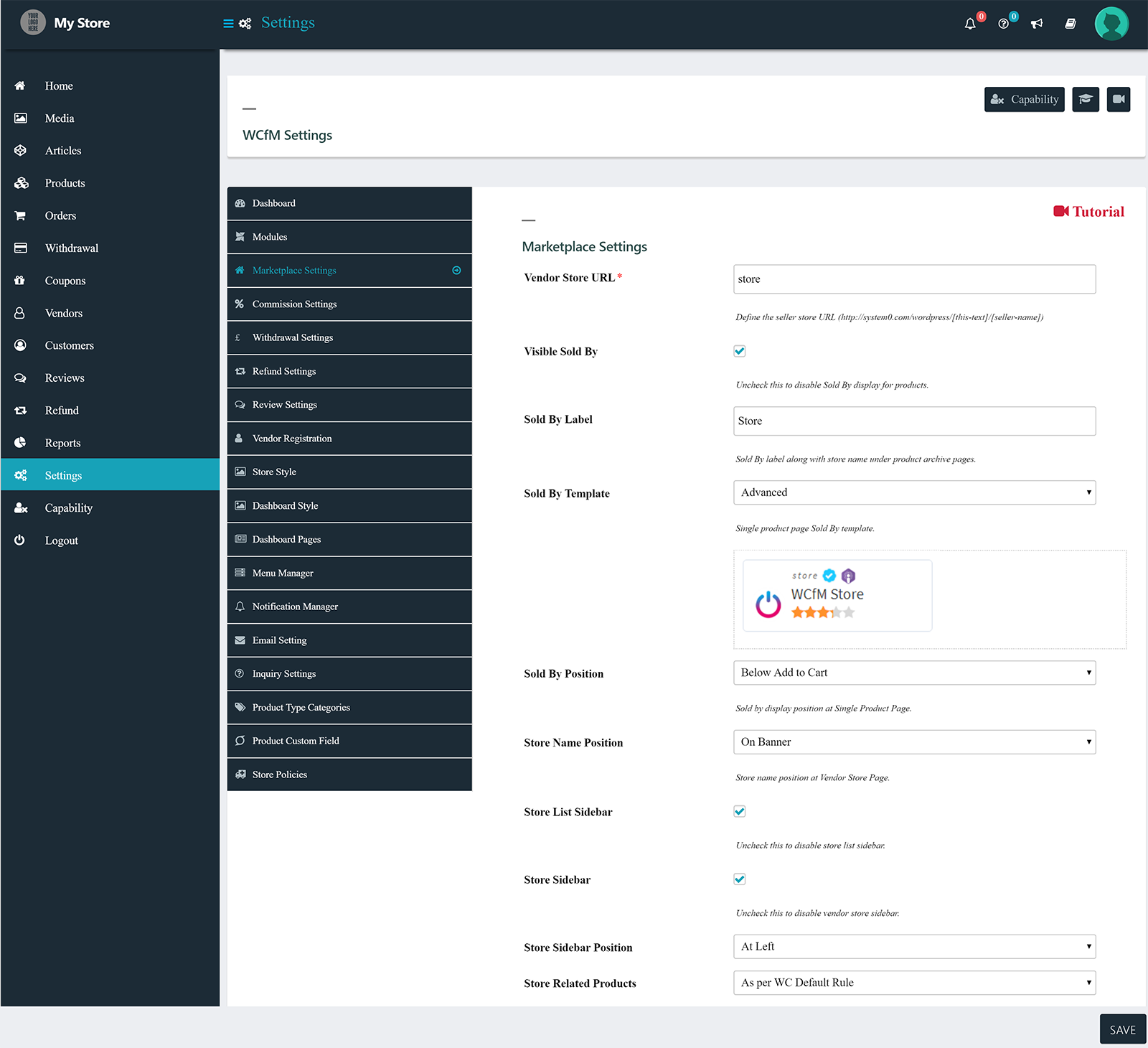**Detailed Caption:**

The image appears to be a screenshot of a website with a dark teal header featuring several icons and navigational elements. In the upper left corner, an icon within a circle is present, though its details are difficult to discern due to the low resolution. Adjacent to this is the text "My Store." Slightly to the right of this, three horizontal lines denote a menu icon.

Further to the right, there is a crescent gear icon in dark teal followed by two vertically aligned circles. The word "Settings" is inscribed next to these icons. To the right of the settings icon, a notification bell with the number '0' in a red circle is visible, alongside a question mark icon within a teal circle. Additionally, a small microphone icon, reminiscent of those used by broadcasters, appears next to an icon resembling a book and a silhouette of a person.

The background of the header has a greenish-teal hue. Below this header, the main section of the website is divided into a left column and a right column. The left column functions as a menu with various options such as Home, Media, Articles, Products, Orders, Withdrawals, Coupons, Vendors, Customers, Reviews, Refund, Reports, Settings, Capability, and Log Out.

The right column showcases the "WCFM Settings" with further interaction options. Next to this title is another icon and a button labeled "Capability." Additional buttons designed like a graduation hat and a camera or video recorder are also present. Below these buttons is a detailed submenu listing items like Dashboard Modules, Marketplace Settings, Commission Settings, Withdrawal Settings, Refund Settings, Review Settings, Vendor Registration, Store Style, Dashboard Style, Dashboard Pages, Menu Manager, Notification Manager, Email Settings, Inquiry Settings, Product Type Categories, Product Custom Fields, and Store Policies.

At the bottom part of the website, there is a gray bar hosting a "Save" button situated in the lower right corner. The website's main interface showcases an interactive form where each field name is accompanied by an input field directly to its right.